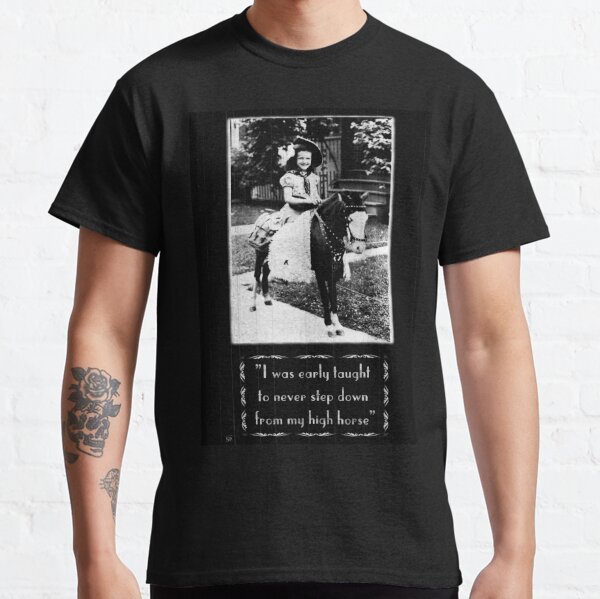A young man, whose face is cropped out, is modeling a short-sleeved, dark grey t-shirt in front of a white wall with a brick pattern. The t-shirt features a rectangular black-and-white vintage photograph on the chest, depicting a young girl riding a pony in front of a house with a stone staircase and grass. Below the image, in an antique-style white border reminiscent of silent movie title cards, are the words: "I was early taught to never step down from a high horse." The man’s right arm is visible, showcasing a detailed tattoo of a skull with a rose entwined around it. The overall image has a slightly noisy, aged appearance, enhancing its nostalgic feel.